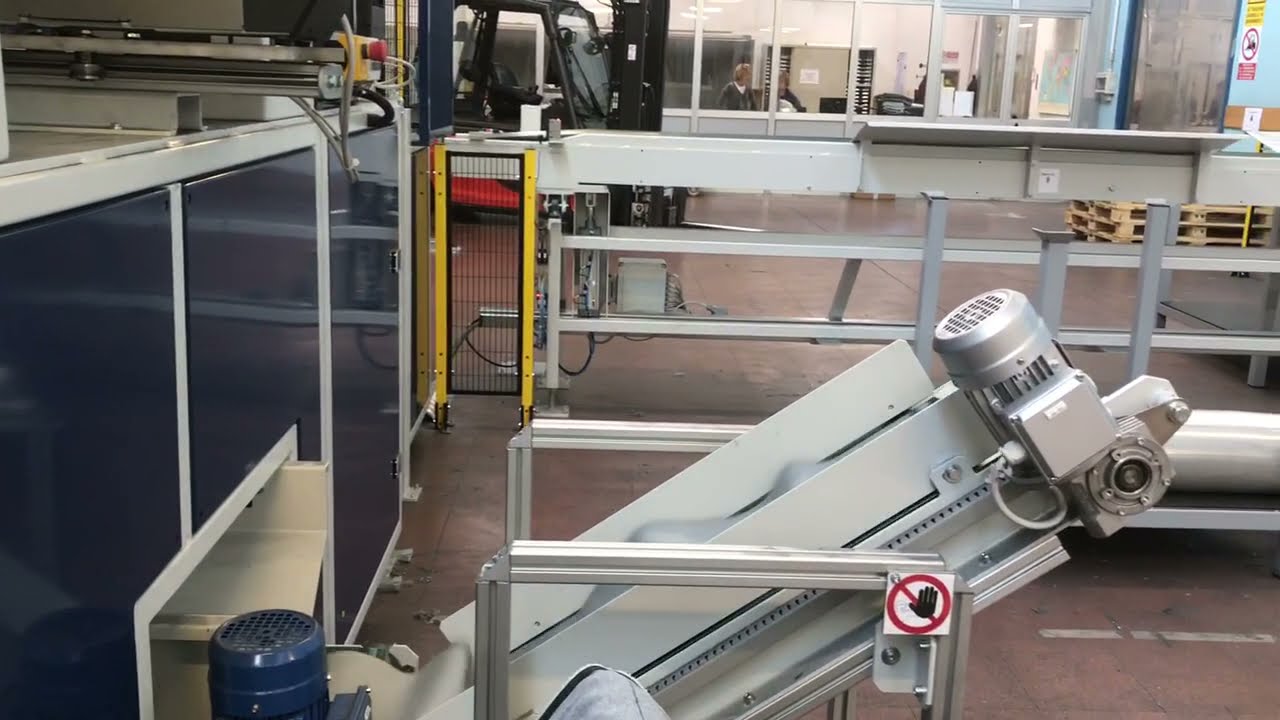The photograph captures an industrial warehouse or factory setting filled with detailed elements and machinery. In the foreground, there's a complex machine, possibly designed for producing candy or food, given the multi-hole extrusion component that leads to a conveyor belt and subsequently into a storage compartment or oven. This machine features a prominent silver head and a large arm, appearing somewhat robotic. Nearby, a warning sign with a circled hand icon suggests a 'do not touch' advisory, indicating safety precautions around the machinery.

The workspace is demarcated by a white metal fence that prevents unauthorized access. Further back, another metallic fence appears, providing an additional safety barrier. Off to one side, there are empty wooden pallets and a pallet distribution machine, indicating this area’s probable use in storage or manufacturing logistics. The floor is tiled in a brownish hue with a shiny surface reflecting overhead lights.

In the background, a black cabinet is visible, situated against the wall, which seems to be connected to the machine. Adjacent to this, windows line the warehouse wall, likely leading to an office space. Through these windows, a couple of people can be seen. Additionally, there's a structure resembling a forklift, identifiable by its pronged bottom and windowed design, further indicating the warehouse nature of the setting.

Overall, the scene is a bustling industrial environment, merging advanced machinery with practical logistics, underscored by stringent safety measures and a complex spatial layout.